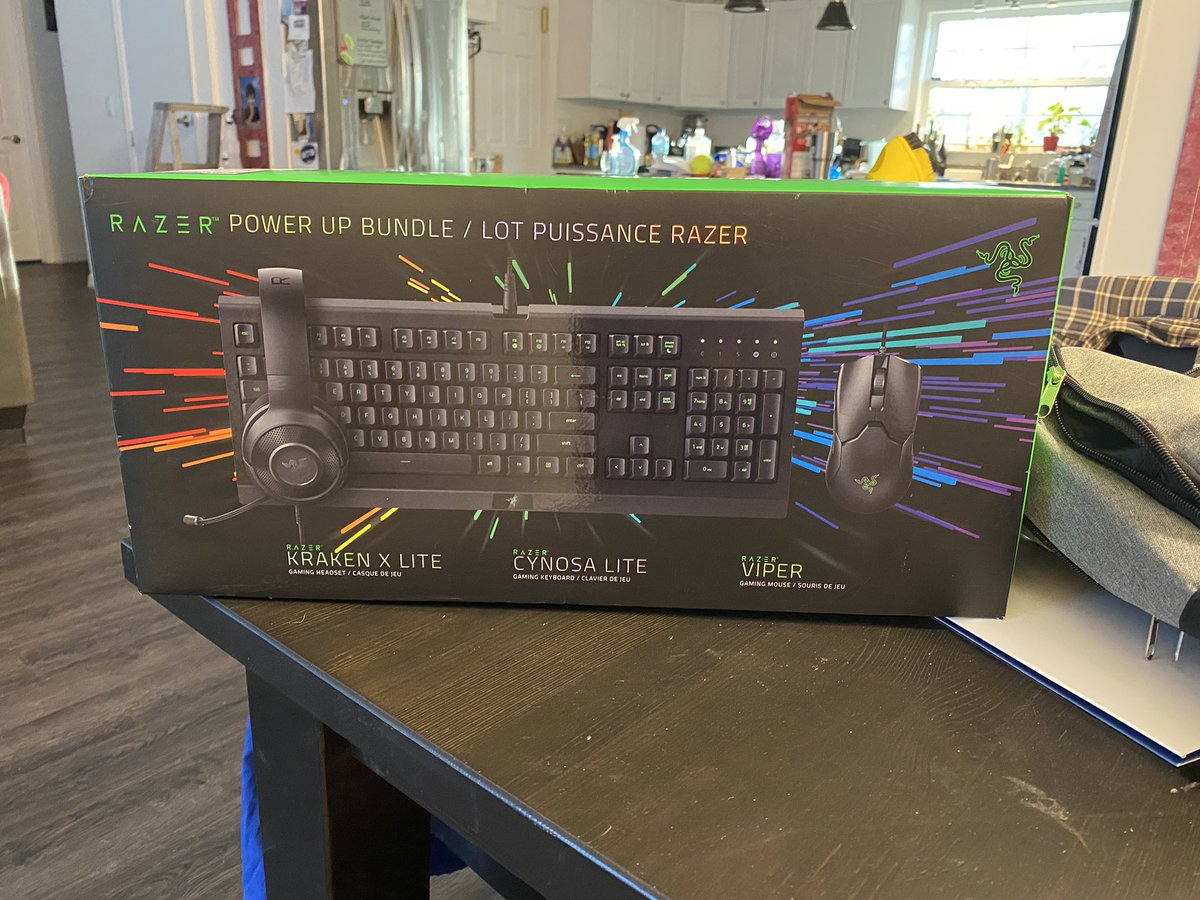The image captures the interior of a home, prominently featuring a brown table at its center. On the table is a rectangular box emblazoned with the text "RAZR Power Up Bundle/Lot Presence RAZR" in bold at the top. The box showcases a sleek black keyboard, a black gaming headset, and a black gaming mouse, all set against the backdrop of their respective product names in both English and French. Specifically, it advertises the "RAZR Kraken X-Lite Gaming Headset," the "RAZR Synosa Lite Gaming Keyboard," and the "RAZR Viper Gaming Mouse."

The background reveals a sunlit kitchen, visible through a window in the far right corner. The kitchen counter is adorned with various items, including a cleaning spray, a possible can opener, a knife block, and similar kitchen utensils. To the far right of the frame, a backpack rests on the counter, and a door—potentially leading to a closet—can be seen in the background. A stainless steel refrigerator, festooned with various attached items, completes the domestic scene.